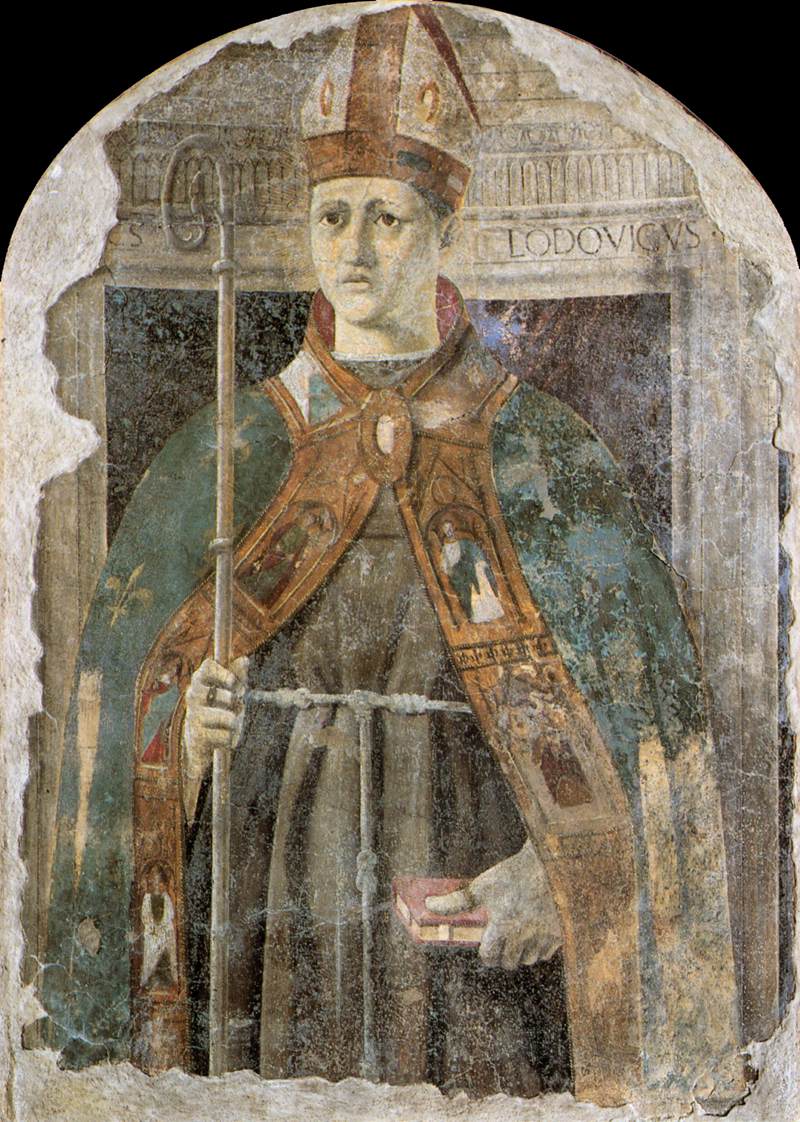This artwork depicts an older, faded painting on an arched, stone-like structure that appears to have been plastered on. The focal point is a religious figure, likely a cardinal or pope, characterized by a tall, red and white hat and a combination of teal, aqua blue, and brown robes, adorned with a white rope tied around the waist. The figure's detailed attire includes a green cloak with fleur-de-lis patterns and portraits of saints, and he holds a red book in his left hand while gripping a long staff with a curled end in his right. The painting is notably aged, with visible chipping and fading, revealing a grayish overtone, and the background features black spaces where the paint has worn away. Accompanying the figure is an engraved gravestone that curves at the top, with additional Greek lettering visible within the image. The cardinal stands solemnly in front of a columned structure, giving the painting a timeless, somewhat somber feel.